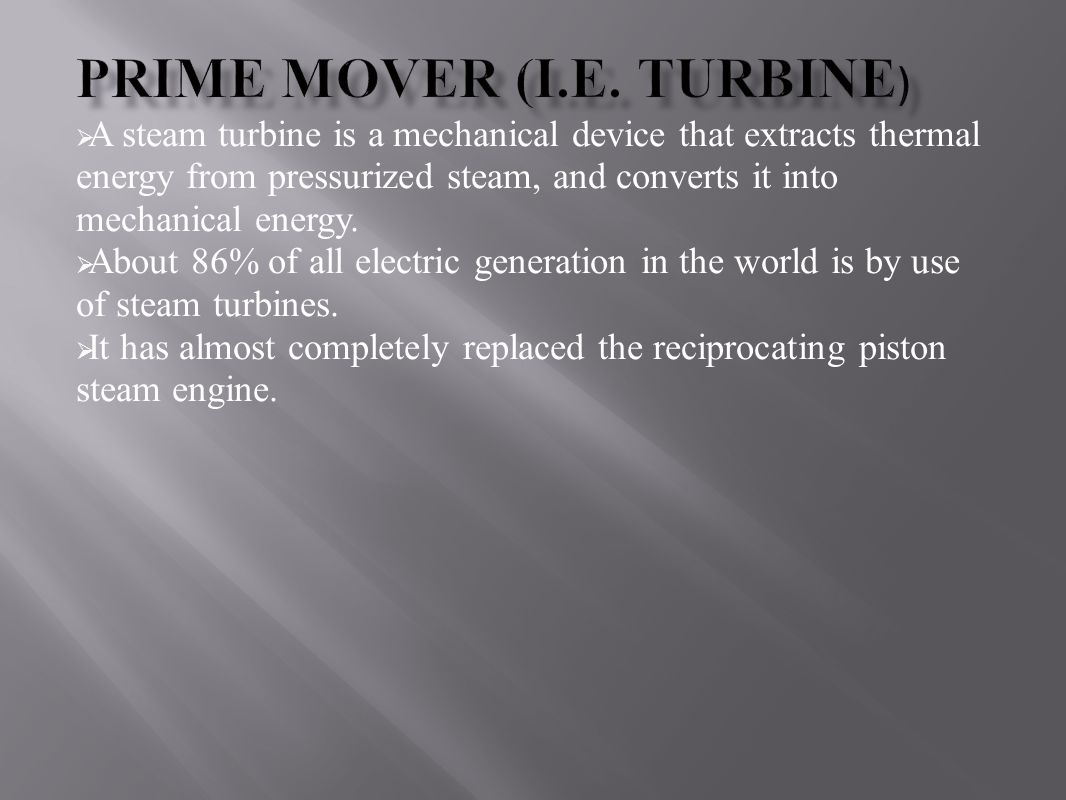This image is a digitally created presentation slide, likely from a PowerPoint, featuring an explanatory graphic about steam turbines. The rectangular slide has a dark gray background with light streaks heading diagonally from the top left to the bottom right, and white striping at the bottom. The title at the top reads "Prime Mover (i.e., Turbine)" in black text with a drop shadow, set in Times New Roman font. Beneath it, in white text, a concise definition states: "A steam turbine is a mechanical device that extracts thermal energy from pressurized steam and converts it into mechanical energy." This is followed by two bullet points: the first one highlights that "about 86% of all electric generation in the world is by use of steam turbines," while the second points out that steam turbines "have almost completely replaced the reciprocating piston steam engine." Each bullet point is marked with a left-pointing arrow, half-gray and half-white, matching the clean, professional style suitable for educational or professional presentations.